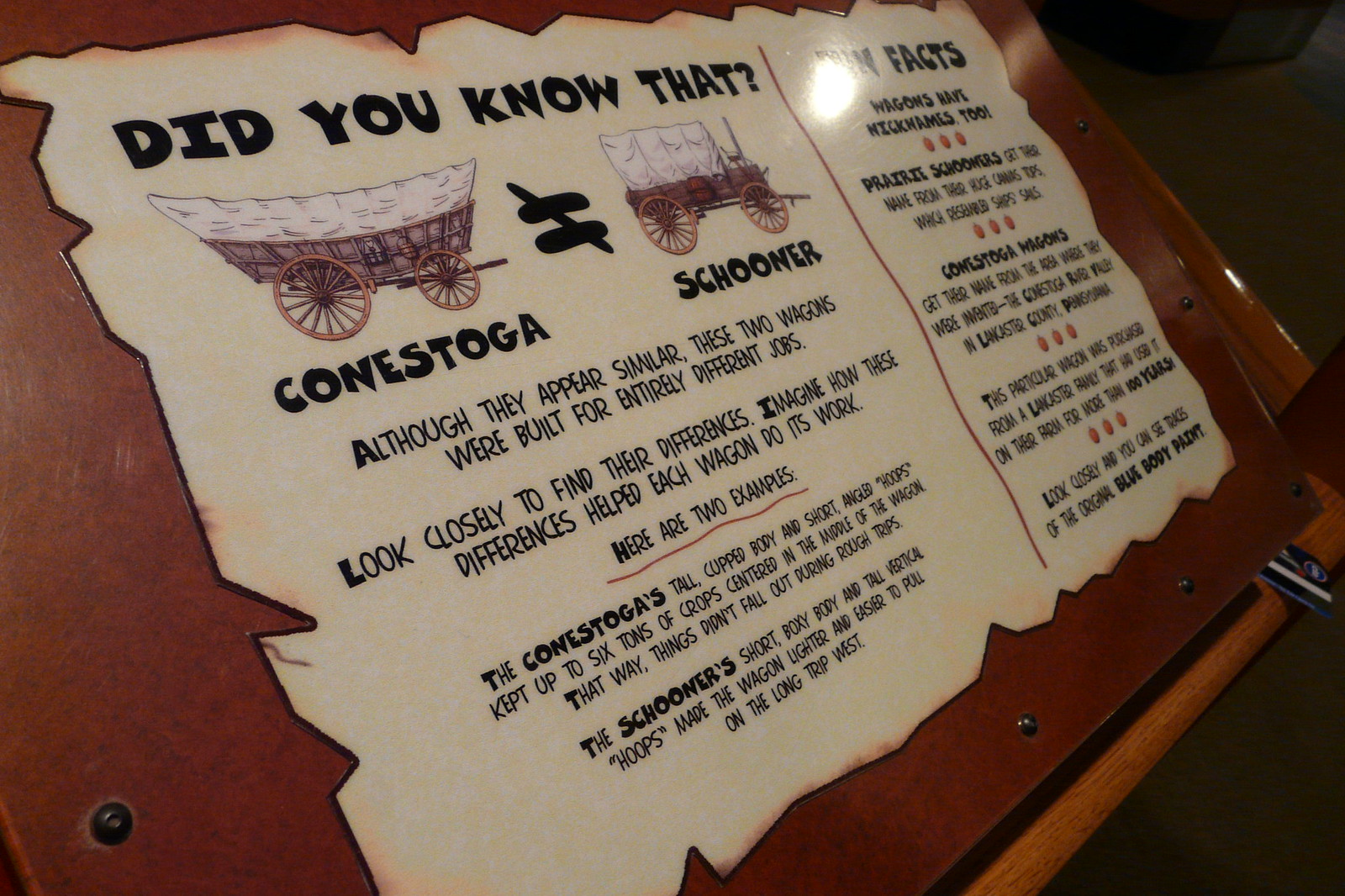This is a detailed museum display on a slanted wooden plaque, featuring two distinct types of horse-drawn wagons: the Conestoga and the Schooner. The display's white background prominently presents the title in large black letters: "Did you know that Conestoga ≠ Schooner?" Above images of each wagon, it explains that although these wagons appear similar, they were built for different purposes. The Conestoga has a tall, cupped body and short, angled hoops to keep up to six tons of crops centered and secure during rough trips. In contrast, the Schooner's short, boxy body and tall, vertical hoops make the wagon lighter and easier to pull on long westward journeys. Below this, a section titled "Fun Facts" lists interesting trivia about wagon nicknames and more. The informative text encourages viewers to observe the differences and imagine how these features helped each wagon perform its specific tasks.